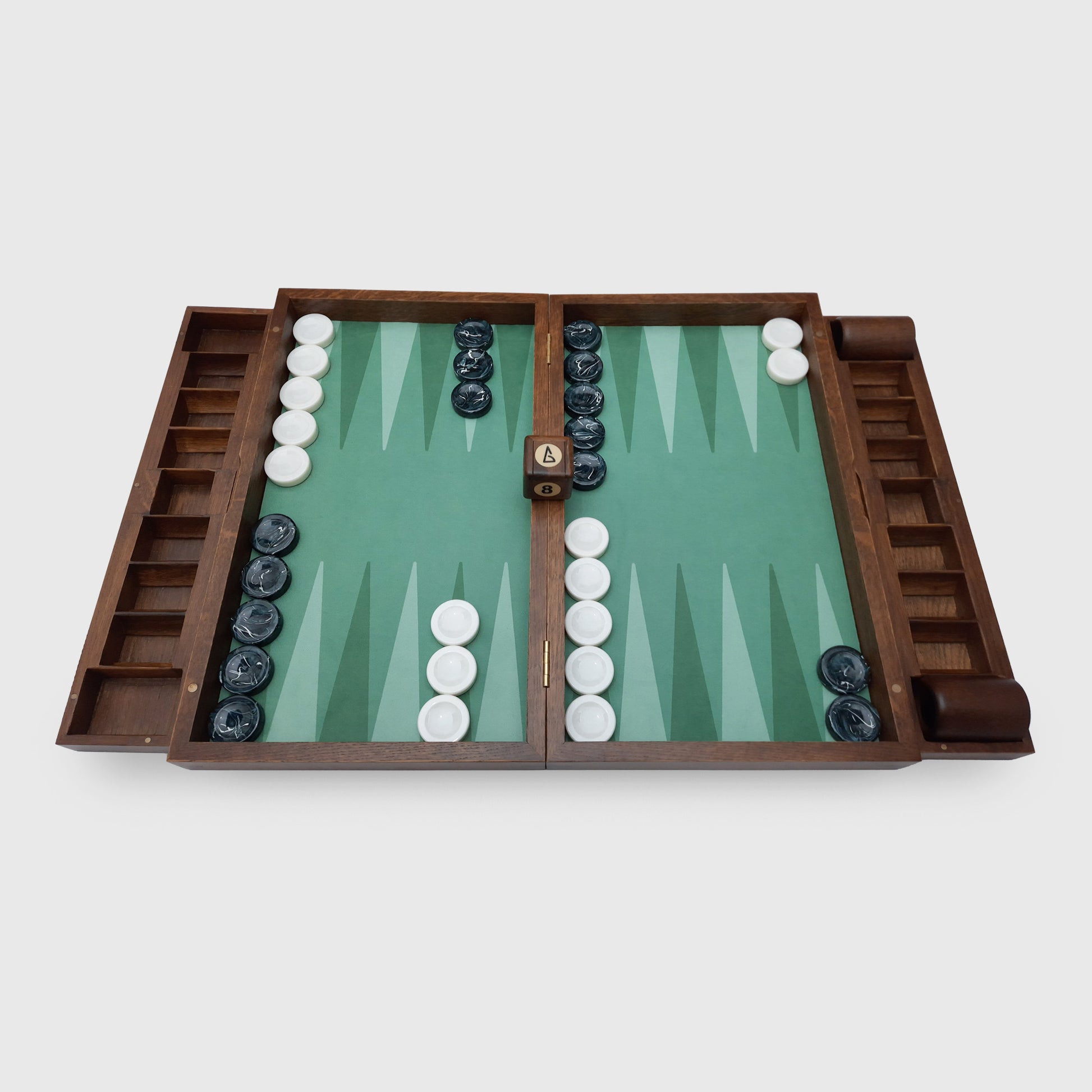This photograph showcases an antique backgammon set against a plain, off-white, light gray background. The focal point is the beautifully handcrafted wooden frame of the board, which features integrated storage pockets on the sides. The board, which is designed to fold up for portability, is opened up to reveal its inner lining of varying shades of green. The main playing surface is a medium green adorned with long triangles in both lighter and darker green hues. White and black playing pieces, resembling checkers, are lined up in rows along the edges. At the center of the board, a wooden die is prominently displayed, adding to the set's vintage charm. This detailed presentation appears to be geared towards a detailed listing, similar to those found on eBay, highlighting the intricate design and classic aesthetic of the backgammon set.